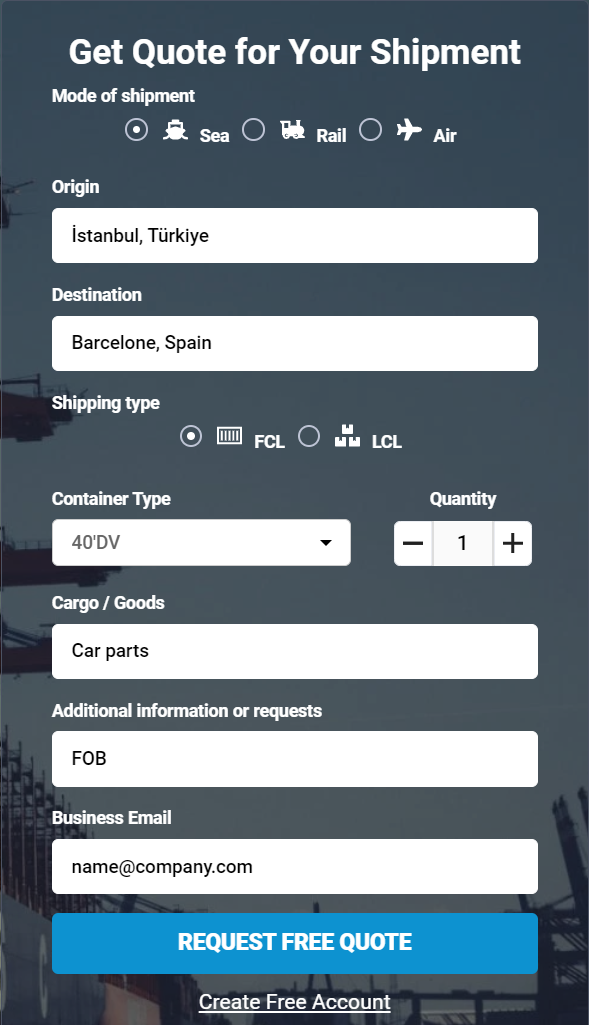**Caption:** 

This image showcases the user interface of a mobile app or website, viewed in portrait mode on a smartphone. At the top of the screen, a white header reads "Get Quote for Your Shipment". Below, there are options for the mode of shipment, featuring selectable radio buttons. The currently selected option is "Sea", highlighted with an image of a boat. To the right, there are additional options: "Rail" accompanied by an image of a train, and "Air" with an airplane icon.

Next, a text box labeled "Origin" displays "Istanbul, Turkey", and beneath it, "Destination" is marked as "Barcelona, Spain". Following this, under "Shipping Type", two radio button options are presented: "FCL" with a barcode image, and "LCL" with an image of three stacked boxes.

Further down, there is a section for "Container Type" showing a dropdown menu currently set to "40 DB" and a specified quantity of one. The "Cargo / Goods" field is filled with "Car parts", and an "Additional Information or Requests" box contains the term "FOB".

Towards the bottom, a field labeled "Business Email" displays "name@company.com". Near the footer, a prominent blue button with white text urges users to "Request Free Quote." At the very bottom, a white link invites users to "Create Free Account."